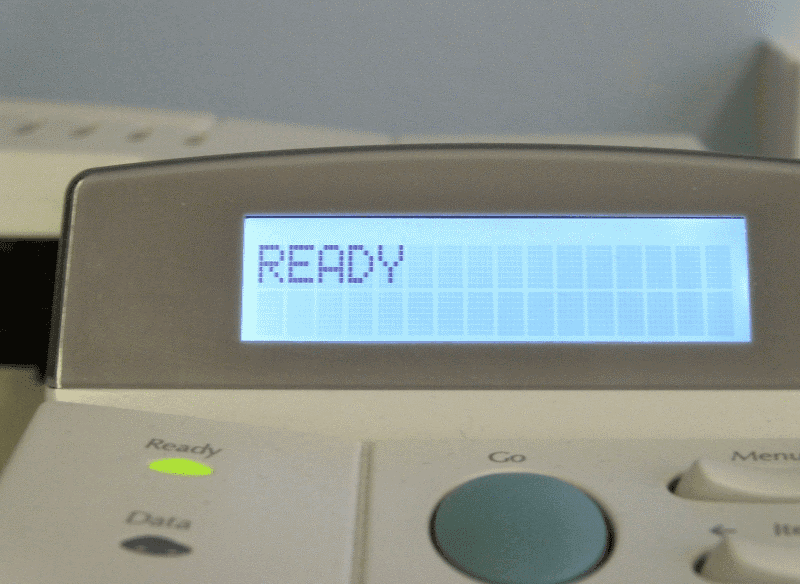This photo is a close-up of a control panel for some sort of device, possibly a piece of machinery or an electronic control system. The background of the panel is a deep gray color, while the main screen is a blue digital display showing the word "READY" in pixelated letters. Below the screen, there are two oval indicator lights: one green light labeled "READY," which is lit, and a gray light labeled "DATA," which is not lit. Towards the front bottom of the control panel, there is a large, round, blue button with the word "GO" above it in black text. To the right of the blue button, there are two vertical push buttons or toggle switches. The top button is labeled "MENU," and the bottom button has an arrow pointing to the left above it, but the text is unclear due to blurriness. The panel's layout suggests various operational controls and indicators, with the primary emphasis on the readiness and data status of the device.